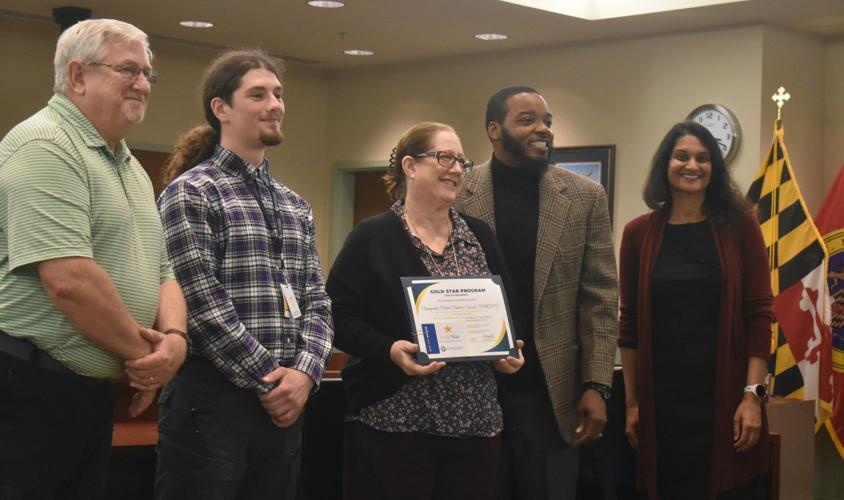In this horizontally aligned rectangular photograph, five people are standing side by side, posing for a picture while looking to their right, where another camera is likely taking their photograph. On the left, a heavyset man in a striped green polo and black pants stands next to a younger man with a brown ponytail and facial hair, dressed in a plaid button-down shirt and black pants. Centrally positioned is a middle-aged woman holding an award, labeled "Gold Star Program," with her hair pulled back in a clip. She wears a black cardigan over a black and white blouse. To her right is a dark-skinned man smiling warmly, dressed in a black shirt and a brown and gold plaid suit jacket. On the far right, a long-haired woman in a red cardigan over a black dress or top is the only one looking directly at this camera. Behind them, light beige walls and recessed ceiling lights suggest an indoor room resembling a courtroom. A silver-framed clock with a white face is mounted on the right wall, near a striped gold and black flag with a small cross on top, flanked by additional flags featuring black and yellow checkered patterns with red and white designs.